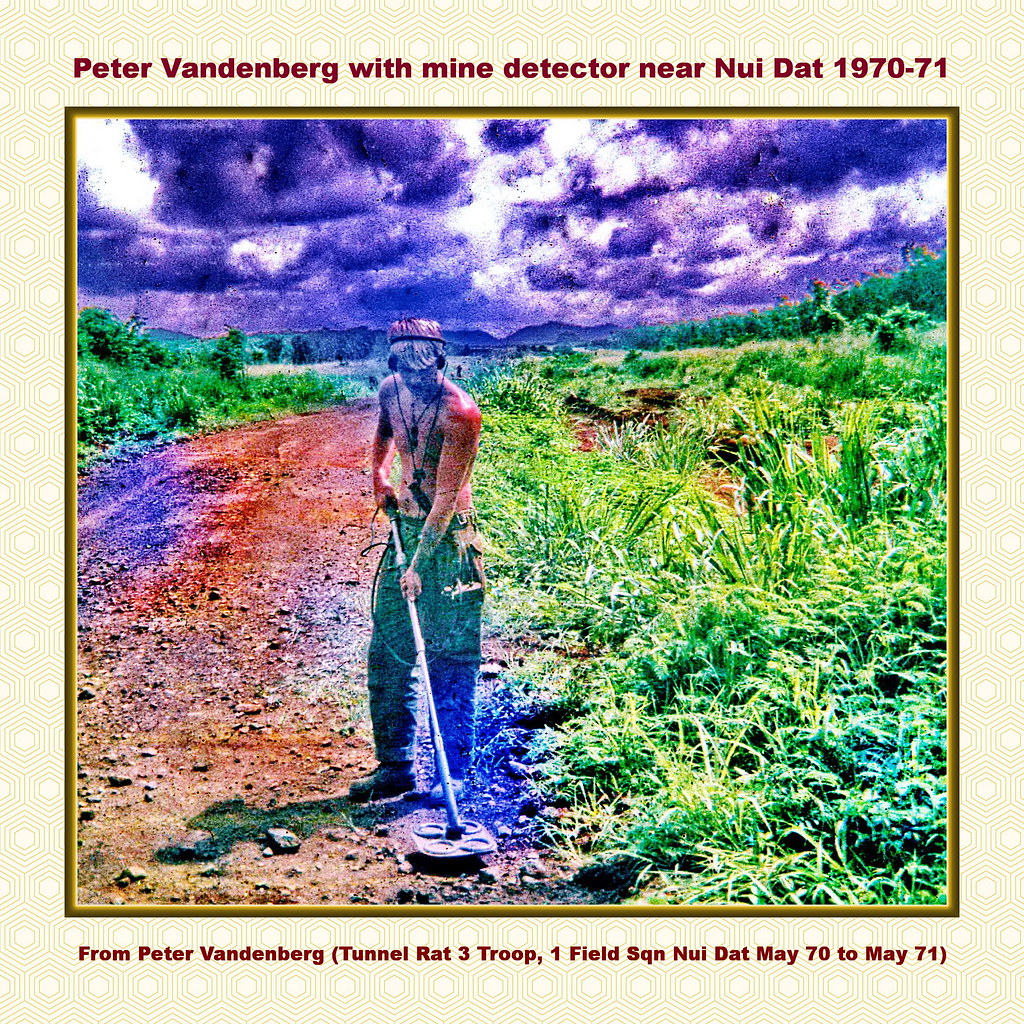This colorized and slightly overexposed square-format photograph from 1970-71 showcases Peter Vandenberg, a shirtless young soldier with short blond hair, standing on a dirt path near Nui Dat. The photograph has a noticeable bluish and reddish tint, likely due to color editing or hand tinting, which gives the clouds a purplish hue and adds unnatural blue patches to the dirt road and surrounding vegetation. Peter, wearing military fatigue trousers and boots, is focused intently on a mine detector he's using, with headphones connected to the device. The background reveals a stormy, menacing sky with dark red clouds and green vegetation on either side of the path leading to blue mountains in the distance. The top of the image is captioned with "Peter Vandenberg with mine detector near Nui Dat, 1970-71," and the bottom reads "From Peter Vandenberg, Tunnel Rat 3 Troop, 1 Field SQN, Nui Dat, May 70-May 71." This detailed depiction captures a moment of tension and vigilance during Vandenberg's service as a Tunnel Rat.